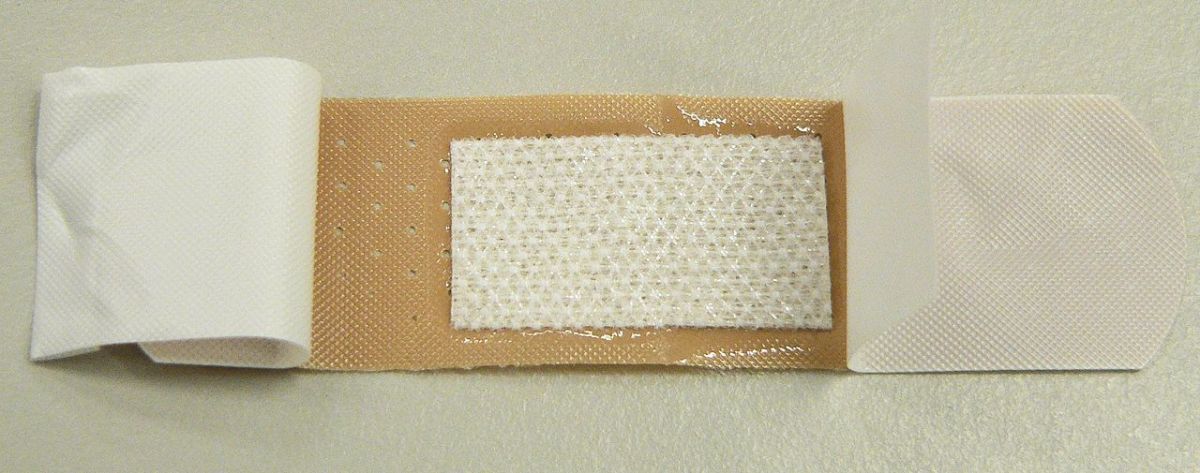The image showcases a new, clean Band-Aid lying flat on a solid beige background. The Band-Aid, facing adhesive side down, is in the process of having its protective plastic backing partly removed. The tan adhesive strip on the left side is pulled back, revealing the white, mesh cloth pad meant for covering wounds, with tiny perforations visible in the adhesive area around it. The right side remains intact, with the tab still in place. The photograph captures a close-up view, highlighting the slightly shiny, pristine condition of the Band-Aid, suggesting it has never been used.